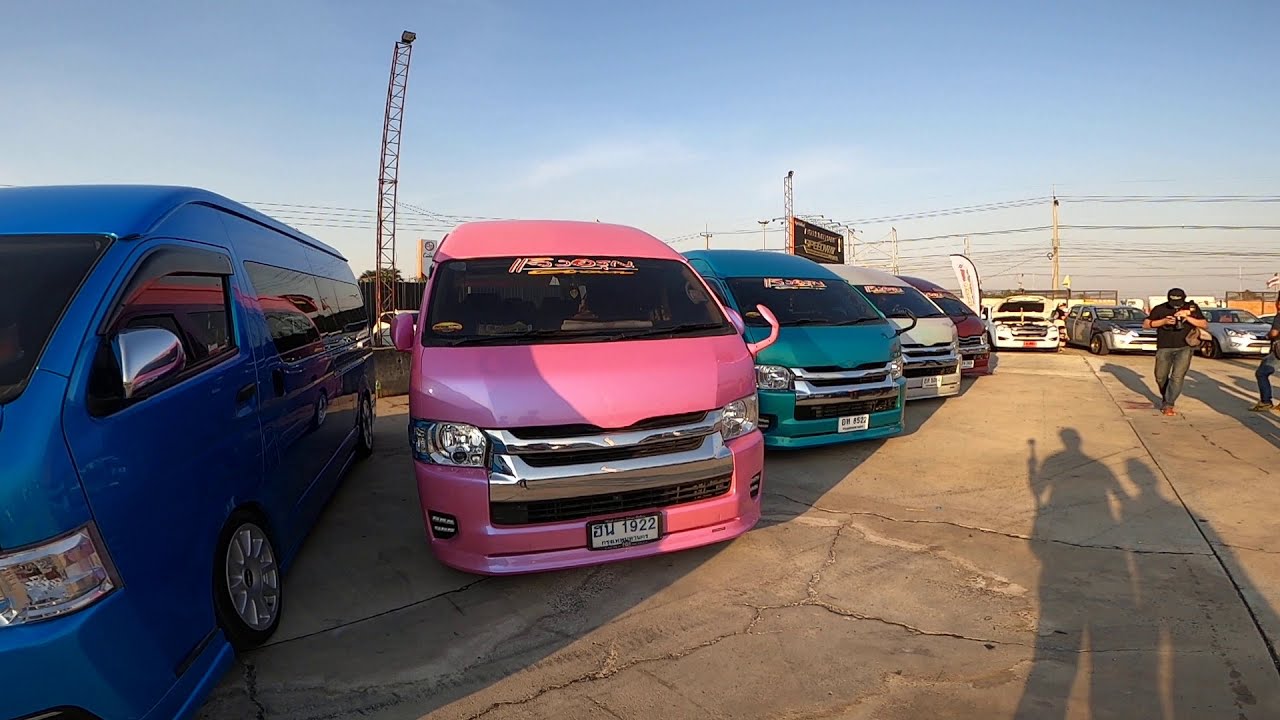The photograph appears to have been taken in a car dealership parking lot located in a foreign country, evidenced by the distinct shape and numbers on the license plates. The image prominently features a row of stylish, boxy vans, arranged at a 45-degree angle on cracked concrete. From left to right, the colors of the vans are a bright bluish-purple, pink, turquoise, white, and red. A man, dressed in a black t-shirt, jeans, and a black baseball cap, is walking towards the camera while looking down. Shadows on the bottom right of the image likely belong to the photographer, who may be holding a GoPro, and another person standing beside them. Behind the row of colorful vans, more vehicles are visible, parked in a straight line. The background features a metal scaffolding structure, resembling a radio tower, a black billboard with white and yellow text, and some power lines.